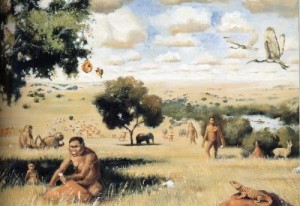In this small, intricate painting depicting early hominid life, a vast grassland landscape stretches under a blue sky laden with white, billowy clouds. The arid scene, dominated by beige and tan hues, is punctuated by patches of lush greenery surrounding a watering hole, providing a sharp contrast to the parched surroundings. Crane-like birds elegantly soar from the right, adding a dynamic sense of movement to the tranquil atmosphere.

Scattered throughout the image, several hominid figures, with distinctive large heads and high cheekbones, engage in various activities. These early humans, with brownish skin tones, are depicted both walking upright and kneeling in the foreground, suggesting a mix of social and survival behaviors. Among them, animals blend into the scene effortlessly—an elephant meanders in the background, while closer to the viewer, a lizard resembling a bearded dragon perches on a rock, basking in the sun’s warmth. Additionally, a beehive hangs from one of the sparse trees, hinting at the varied ecosystems existing within this prehistoric tableau.